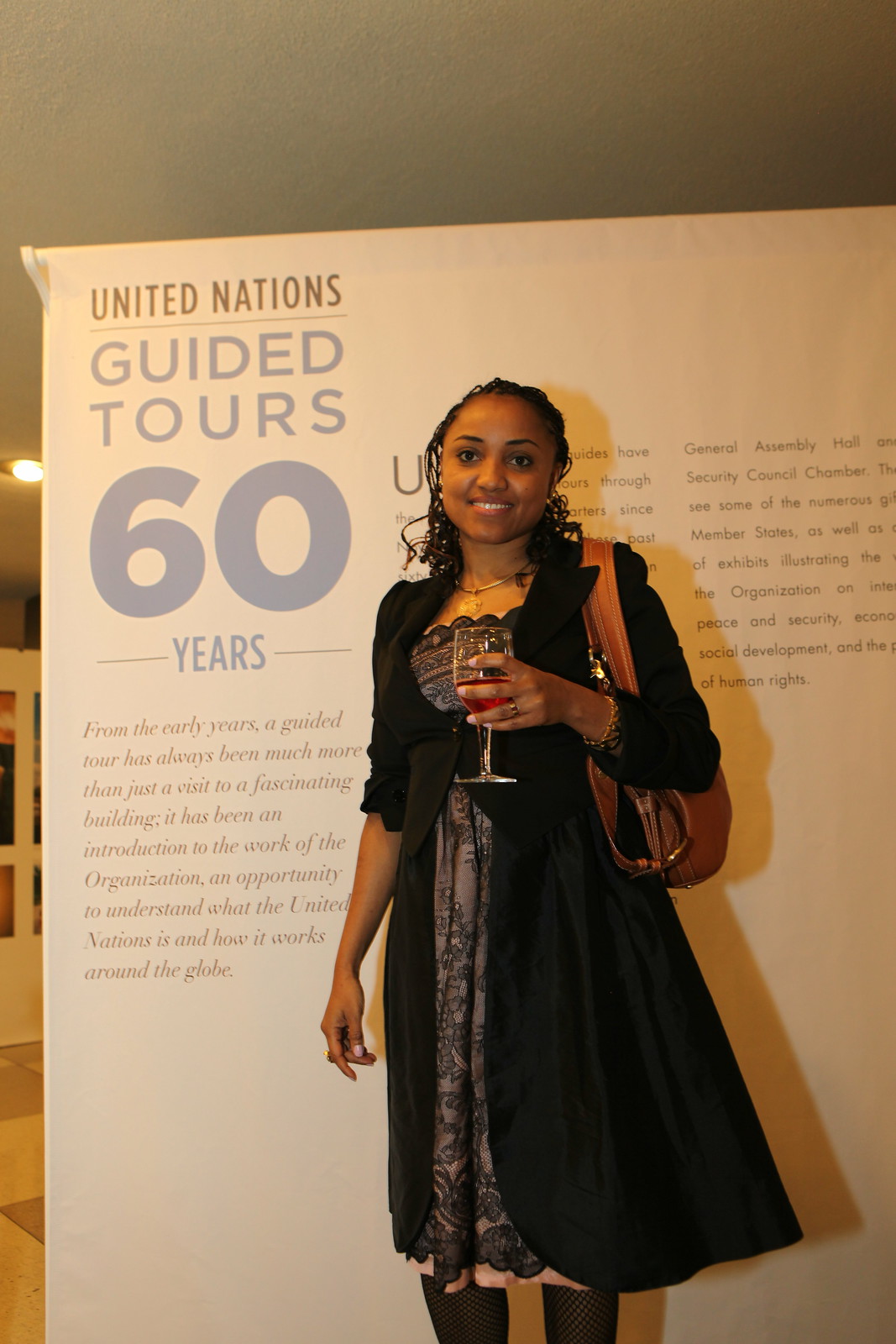The image captures a young black woman standing confidently in front of a large white sign at an interior location with slightly yellow lighting. She is smiling warmly at the camera, her black hair styled in micro braids that are pulled back at the top while the rest cascades down to her shoulders. Dressed elegantly, she wears a long black lace dress with a grey center and a black knee-length coat over it. In her left hand, she holds a wine glass filled with rosé wine, and her right arm rests naturally by her side, adorned with a light brown leather handbag over her left shoulder.

The prominent sign behind her reads “United Nations Guided Tours 60 years” in black and blue lettering at the top left corner. Below it is a legible paragraph that provides an insight into the essence of these tours; it states that from the early years, a guided tour has always been more than just a visit to a fascinating building. It introduces visitors to the world of the organization and offers an opportunity to understand what the United Nations is and how it operates globally. Further to the right side, another readable paragraph mentions the “General Assembly Hall, Security Council Chamber,” and refers to numerous exhibits illustrating the organization's member states and activities. Additional elements like the ceiling and a white divider are visible in the background, emphasizing the indoor setting.